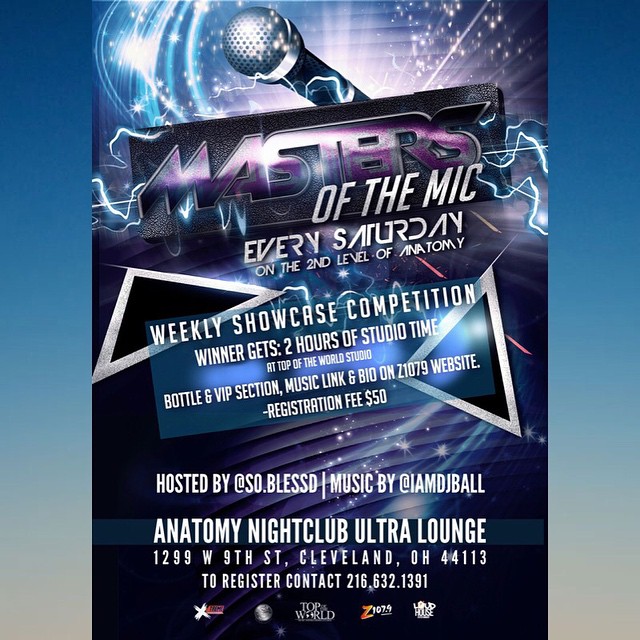The advertisement features a dynamic and colorful design fading from dark blue to a lighter hue, creating an effect reminiscent of a sunrise. The central area of the ad includes gradients of white, blue, and a touch of purple, with several striking graphical elements. At the top, a prominently displayed microphone with a silver band and dark top is illuminated by a light source. Around the microphone, there are several bright, space-like images similar to fireworks, along with a mix of curved white lines and straight rays of light on the right side, transitioning from purple to blue.

Below, a black rectangle shoots out white lightning lines to the left and right. The text "Masters" in purple letters is featured above "Of the Mic" in white letters. Further down, it states, "Every Saturday on the second level of Anatomy," accompanied by a geometric design of two right-angled triangles, one on the left with its hypotenuse facing downwards, and one on the right with the hypotenuse pointing slightly upwards and to the right.

The promotional details include: 
- "Showcase Competition"
- "Winner gets two hours of studio time at the Top of the World studio"
- "Bottle and VIP section"
- "Music link and bio on Z1079 website"
- "Registration fee, $50"

The advertisement also highlights the hosts: 
- "Hosted by @SO.BLESSD"
- "Music by @IAMDJBALL"

At the bottom, venue details are provided:
- "Anatomy Club, Ultra Lounge, 1299 West 9th Street, Cleveland, Ohio, 44113"
- "To register, contact 216.632.1391"

There are small, somewhat harder-to-read logos at the bottom, including "Top World" and "Z1090." The colorful and electrifying design, with sparkles and shiny triangular shapes, stands out against alternating bands of purple and black.